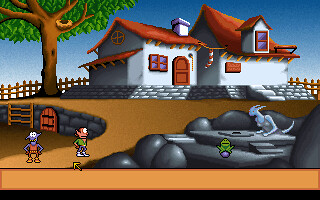The image is a small screenshot from an old vintage point-and-click computer game designed for children, characterized by its cartoony, cute, and slightly pixelated art style. At the center of the scene is a tannish-brown hilltop, atop which sits a quaint white house. The house features a door, several windows, and charming orange-sloped roofs. To the left of the house stands a tree with a robust brown trunk and lush green foliage. At the base of the hill, a couple of small, roughly humanoid characters with pointy ears can be seen. On the right side of the image, there is an altar surrounded by boulders, and it appears to be accompanied by a dragon, adding a touch of fantasy to the scene.